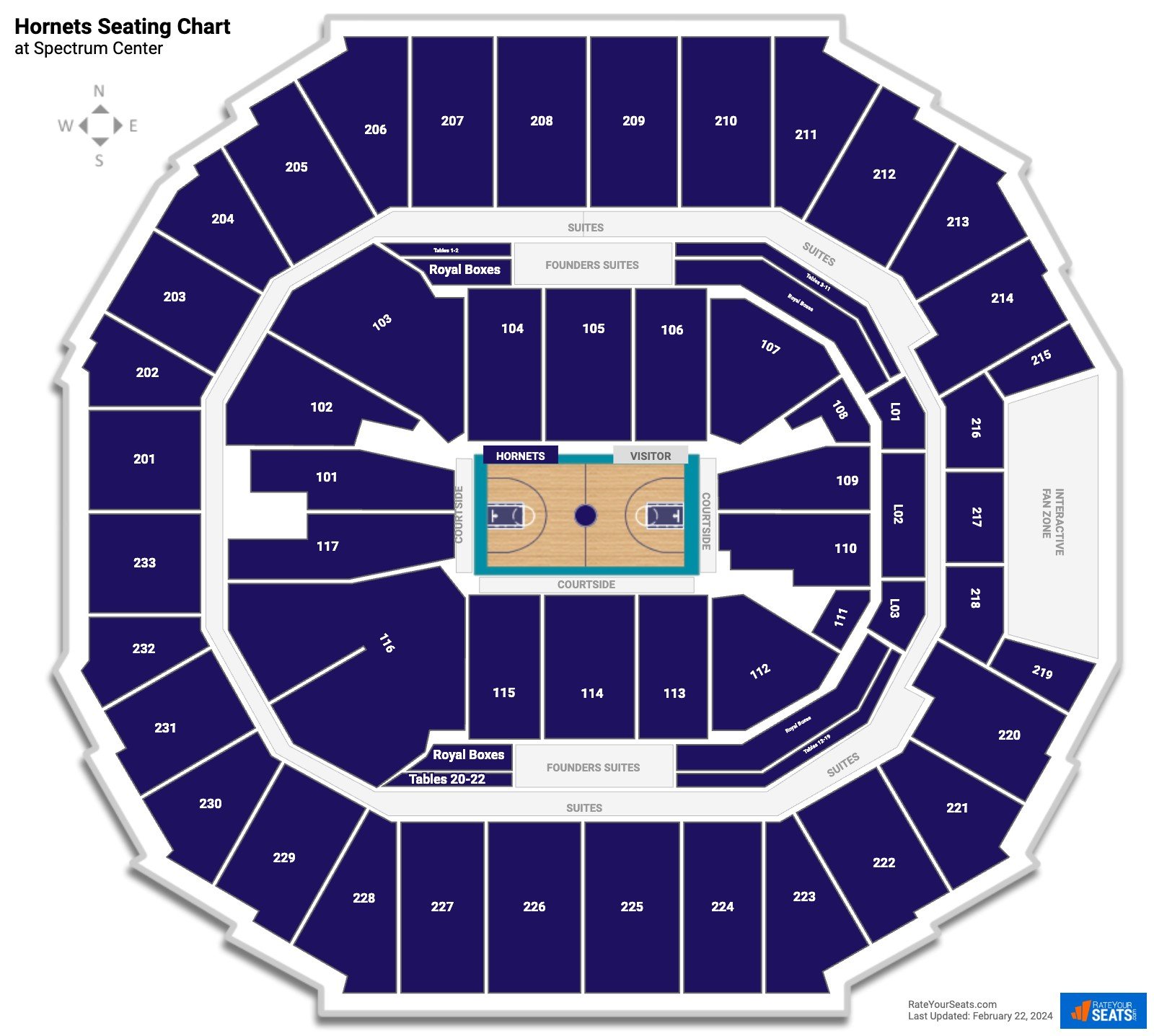A detailed seating chart for the Hornets at the Spectrum Center. At the top left of the image, in bold and larger text, it reads "Hornet Seating Chart," followed by "Ed Spectrum Center" in smaller text beneath it. Dominating the image is the seating layout with a central focus on the basketball court. The court itself is labeled, with "Hornets" on the left in dark blue, and "Visitor" on the right in gray. Encircling the court is a teal-colored perimeter. Surrounding the court are distinct seating sections. Closest to the court is an initial ring of seating, followed by a secondary ring of seating sections set farther back, divided by a white ring designated as "Suites." Each seating section is numbered in white against a dark blue background, making it easy to identify each area.